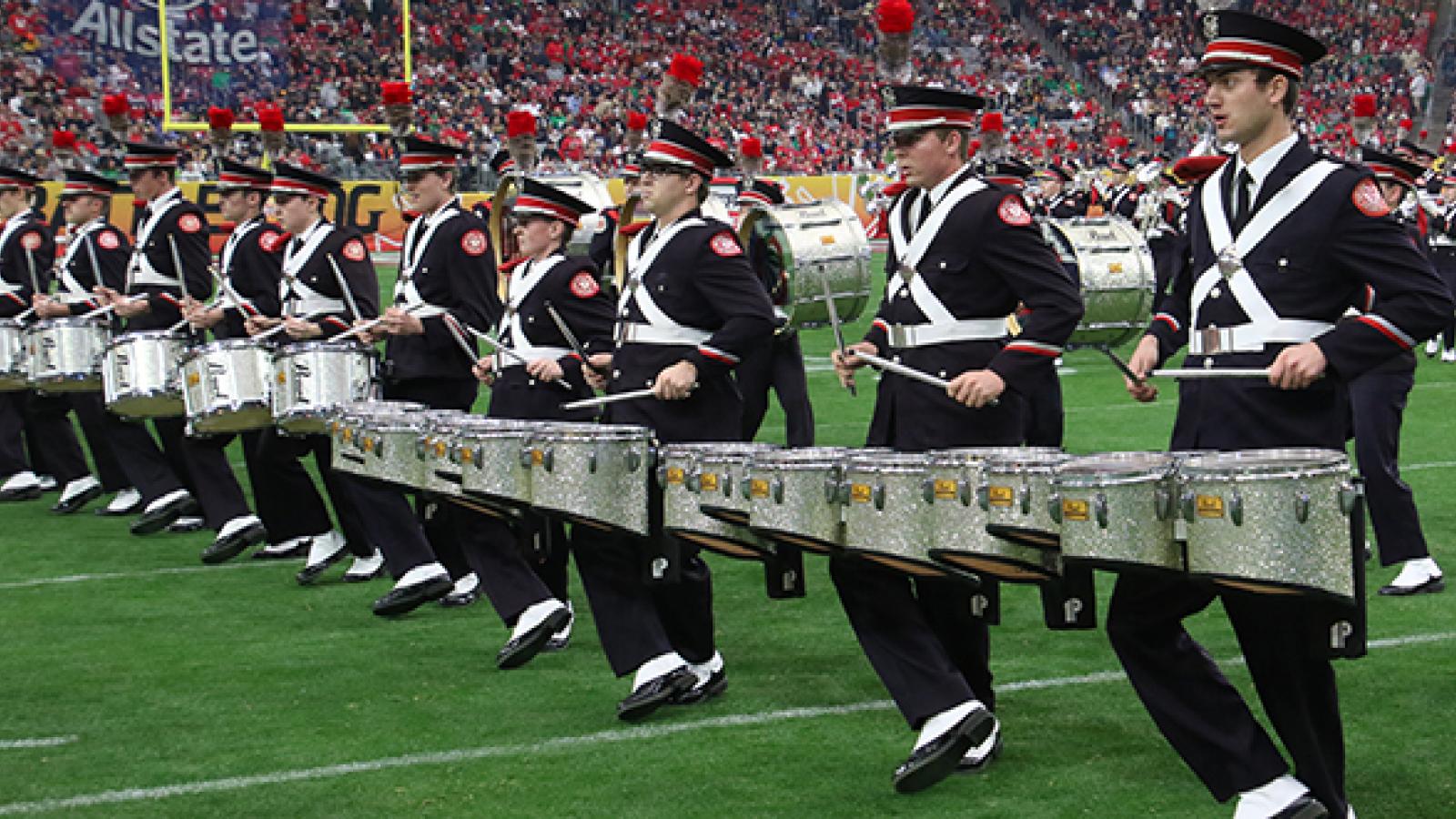This photograph captures a vibrant halftime performance at a packed football stadium, indicated by the completely full seats and the yellow goal post visible in the end zone. The field, typically reserved for American football, is momentarily transformed into a stage for a large group of performers, predominantly drummers, who are outfitted in striking, military-inspired uniforms. They wear black pants, and their drums are secured by white harnesses that form an X across their chests, complemented by black and white shoes. The performers sport black hats adorned with a distinctive red and gold band, adding a touch of color to their coordinated attire.

The drummers, numbering around 20 to 30, are engaged in an energetic routine, characterized by synchronized movements where their left foot is crossed in front of their right, almost as if they are dancing while playing. Some carry a single large drum, while others manage two drums attached at their waist. Behind the front row of drummers, larger drums and additional performers create a complex and dynamic backdrop.

Adding to the festive atmosphere, the crowd—their enthusiasm palpable—contributes to the visual spectacle with red balloons and pom-poms dotting the air, and many spectators donning red attire. An advertisement for Allstate is prominently displayed within the stadium, further anchoring the scene in a contemporary, commercial context.